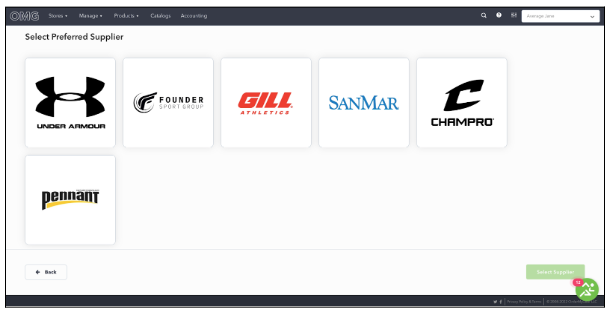This is an image of a computer screen displaying a webpage. At the top of the page, there is a black bar with white, somewhat blurry text that reads "OMG." There are five dropdown menus within this bar, although the text is difficult to read. On the right side of the black bar, there are several icons and a white rectangular dropdown box.

At the bottom of the page, there is a back button located on the left. In the bottom right corner, there is a green rectangular button labeled "Supplier," next to a small green icon depicting a running man and a smaller pink icon with a number inside it.

The main section of the page is titled "Select Preferred Supplier," and features a list of six different supplier options displayed in a white box. The listed companies are: 

1. Under Armour
2. Founder Sport Group
3. Gill Athletics
4. Sanmar
5. Champ Pro
6. Pennant (which is placed alone in the second row)

Each option represents a different company from which one can select their preferred supplier.